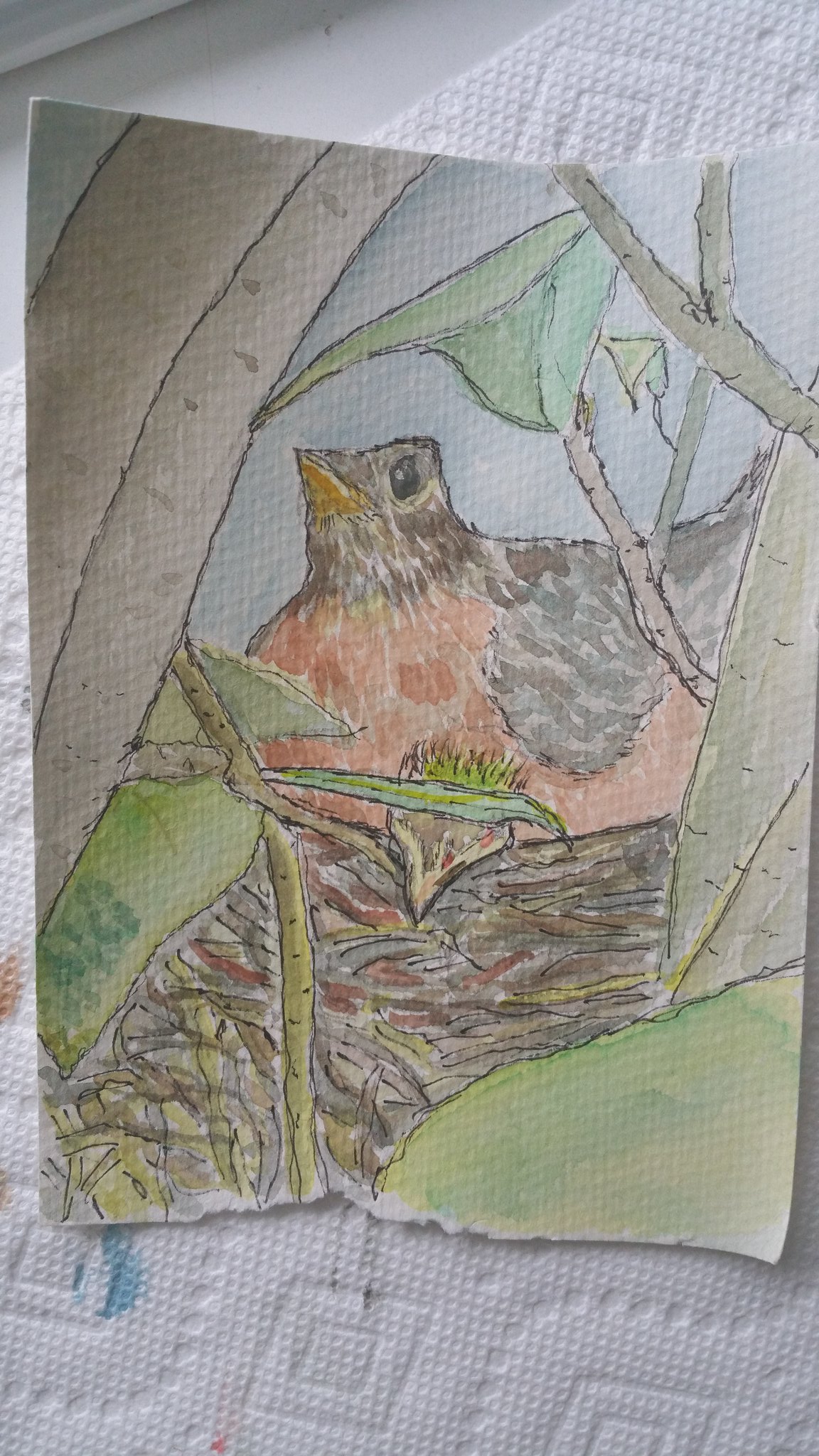A small piece of napkin or paper rests atop a larger napkin, displaying an intricately detailed artwork. The image depicts a robin nestled in its intricately woven nest. The bird is primarily outlined in pen with its internal details masterfully rendered in watercolor. A branch with green leaves extends overhead, providing a canopy under a sky painted in tranquil blue hues. The robin's chest is a vibrant red, contrasting its otherwise brown plumage. Its beak is a bright yellow, and a solitary black eye gazes outward. Nearby, a large leaf dangles from a branch that extends downward to the southeast, partially obscuring the scene. The nest itself is a complex mix of browns, reds, and yellows, adding texture and depth. Just beneath the robin, the head of a baby bird peeks out, while another branch extends from the bottom left corner of the composition. Surrounding the upper left portion of the page are additional brown circles, adding an abstract touch to this charming nature vignette.